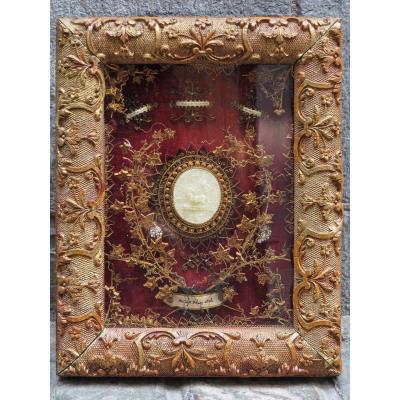This photograph captures a richly detailed framed object displayed against a grayish, potentially concrete wall. The frame is a substantial, heavy-looking wooden structure with an elaborate leaf pattern design and a grainy texture, exhibiting shades of beige to brown, resembling gold in some views. The centerpiece within this ornate frame is strikingly circular or slightly oval and surrounded by intricate blue and brown designs. The object itself, which resembles a medal or brooch, appears silver in color with a decorative border. The background of this central object is a dark red or purplish-red hue, adding depth and contrast to the overall display. Additionally, the display includes three small jewelry pieces above the main object and a plaque positioned below it, further enhancing its museum-like presentation.